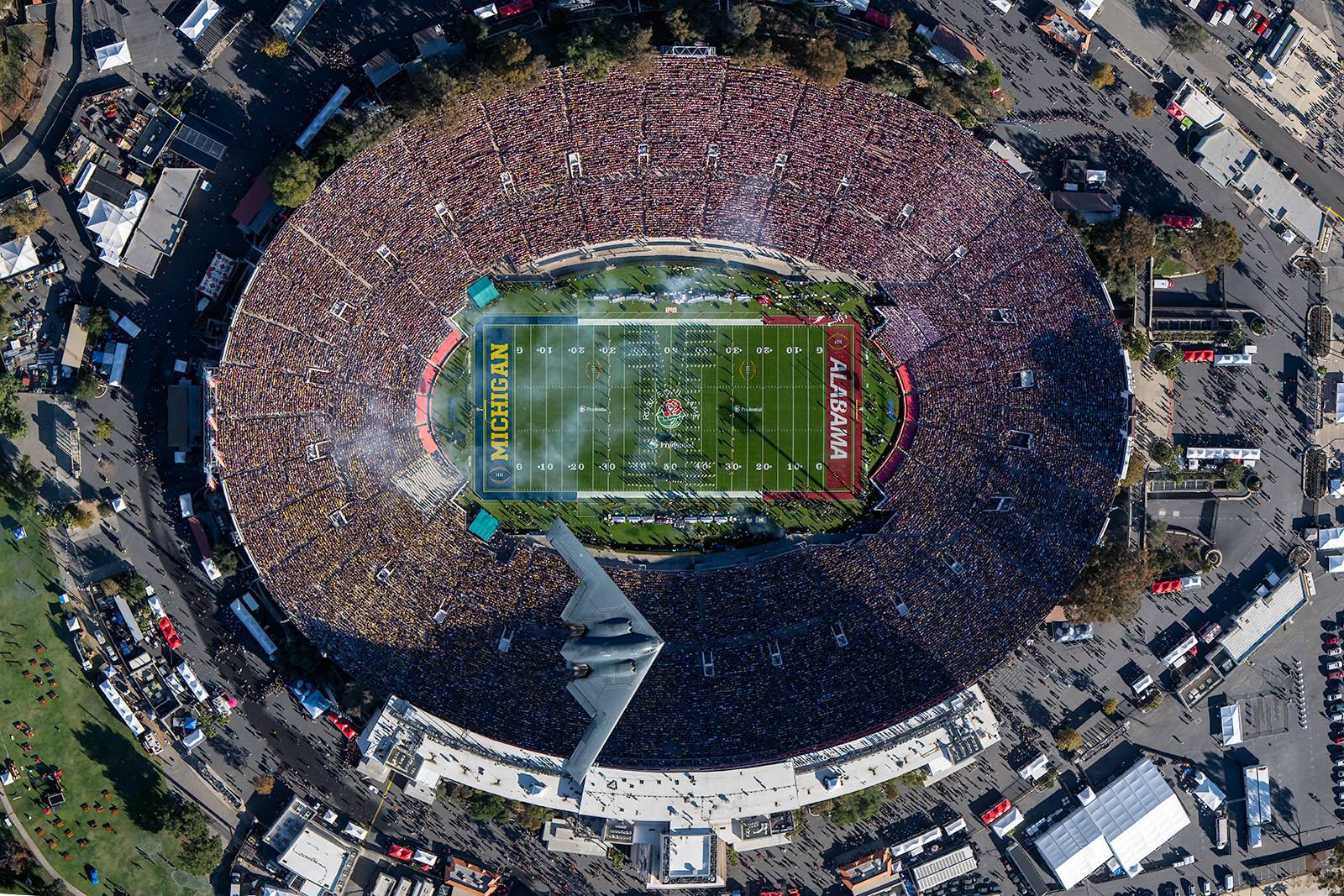The photograph captures an aerial view of a bustling football stadium set in an outdoor, high-altitude location. The stadium, likely hosting a high-stakes bowl game between Michigan and Alabama, is packed to the rafters with spectators, leaving no empty seats in sight. The vividly green football field prominently displays "Michigan" in the left end zone and "Alabama" in the right, with the teams' colors adorning their respective sections. Overhead, a sleek black fighter jet or stealth bomber is soaring, adding a dramatic exclamation point to the event. Surrounding the round stadium, the scene includes numerous parked cars, buses, serene patches of greenery, and scattered groups of people who resemble tiny specks from this vantage point. Nearby buildings and trees also contribute to the detailed, expansive landscape surrounding this exhilarating sports spectacle.